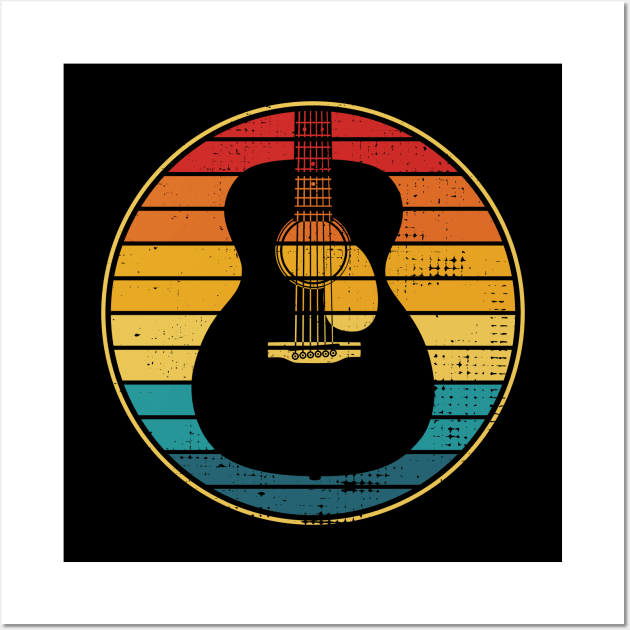The image comprises a striking digital art piece featuring a black acoustic guitar silhouette centered within a yellow circle. The guitar, with visible white strings and a hole through which the colorful background can be seen, stands upright, facing us. Behind the guitar, horizontal stripes fill the circle with shades transitioning from red at the top, to orange, yellow, lighter yellow, light blue, and cyan at the bottom. This circle is then set against a black square backdrop, creating a framed, logo-like appearance. This black square is placed on a white background, and the overall aesthetic gives an intentionally aged or vintage feel.